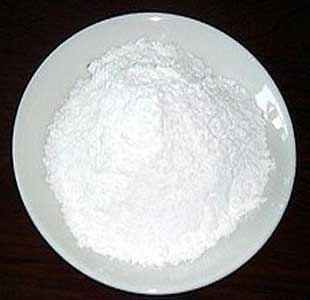This high-angle, photographic image captures a striking scene of a flower-like mound of powdered substance, possibly flour or powdered sugar, sitting elegantly within a shiny, white ceramic dish. The dish, possibly porcelain, features multiple reflections, including a distinct reflection of a window and additional light sources on the top center and bottom center, highlighting its glossy surface. The background is a deep, dark brown, which contrasts sharply with the pristine whiteness of the dish and the mound. The powder is arranged in a triangular shape, elevating in the middle and spreading symmetrically downward, reminiscent of a small mountain. Despite its artistic simplicity, the image is devoid of any contextual clues or text, leaving a sense of intrigue about the scale and setting.